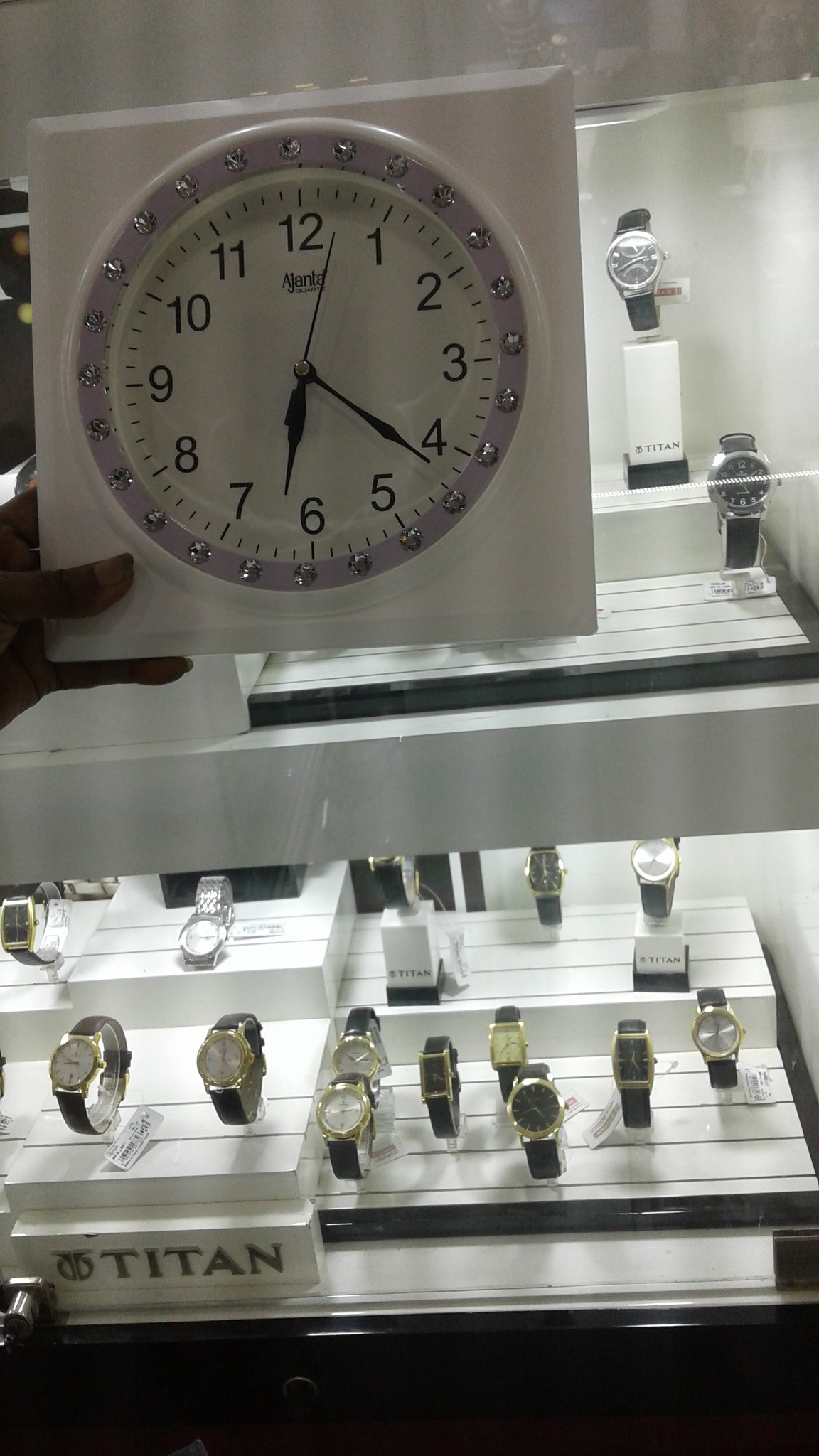In the image, the focal point is a clock inside a white square case. The clock features a purple circular border adorned with small steel rivets. It has three black hands and simple, bold black numbers. The brand name "Alambo" is displayed at the top of the clock face. The clock is being held up by a hand just off-screen to the left, set in front of a glass display case. This case prominently features the gold text "Titan" on a white plaque. Inside the display case, numerous watches are meticulously arranged on white trays with black lines. The watches vary in design—some have circular faces while others are rectangular, with many sporting gold borders and black bands. One tray holds seven watches, another has two, a third in the back contains one silver watch, and a fourth holds three watches. The photograph captures a well-organized assortment of timepieces, suggesting a store setting.